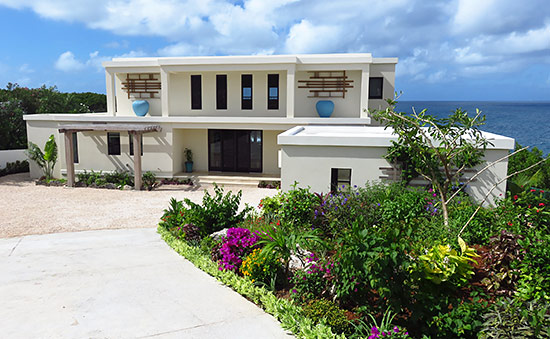The image depicts a luxurious, modern, two-story white cement house with black double glass doors framed by large, vertically rectangular windows on the second floor. The house, situated near a vast and clear blue ocean, showcases an elegant combination of white and cream colors with light tan support pillars on both levels. A light concrete driveway leads up to a light brown stone patio area. The left side of the driveway is lined with lush green shrubs accented with vibrant flowers in hues of yellow, pink, purple, and white, adding a tropical feel to the scene. Two prominent blue flower pots adorn the upper floor windows. The house is partially framed by trees on the left, with puffy clouds and blue sky enhancing the bright, inviting atmosphere. The overall design of the house is modern, square, and aesthetically pleasing, making it an ideal spot for a vacation.